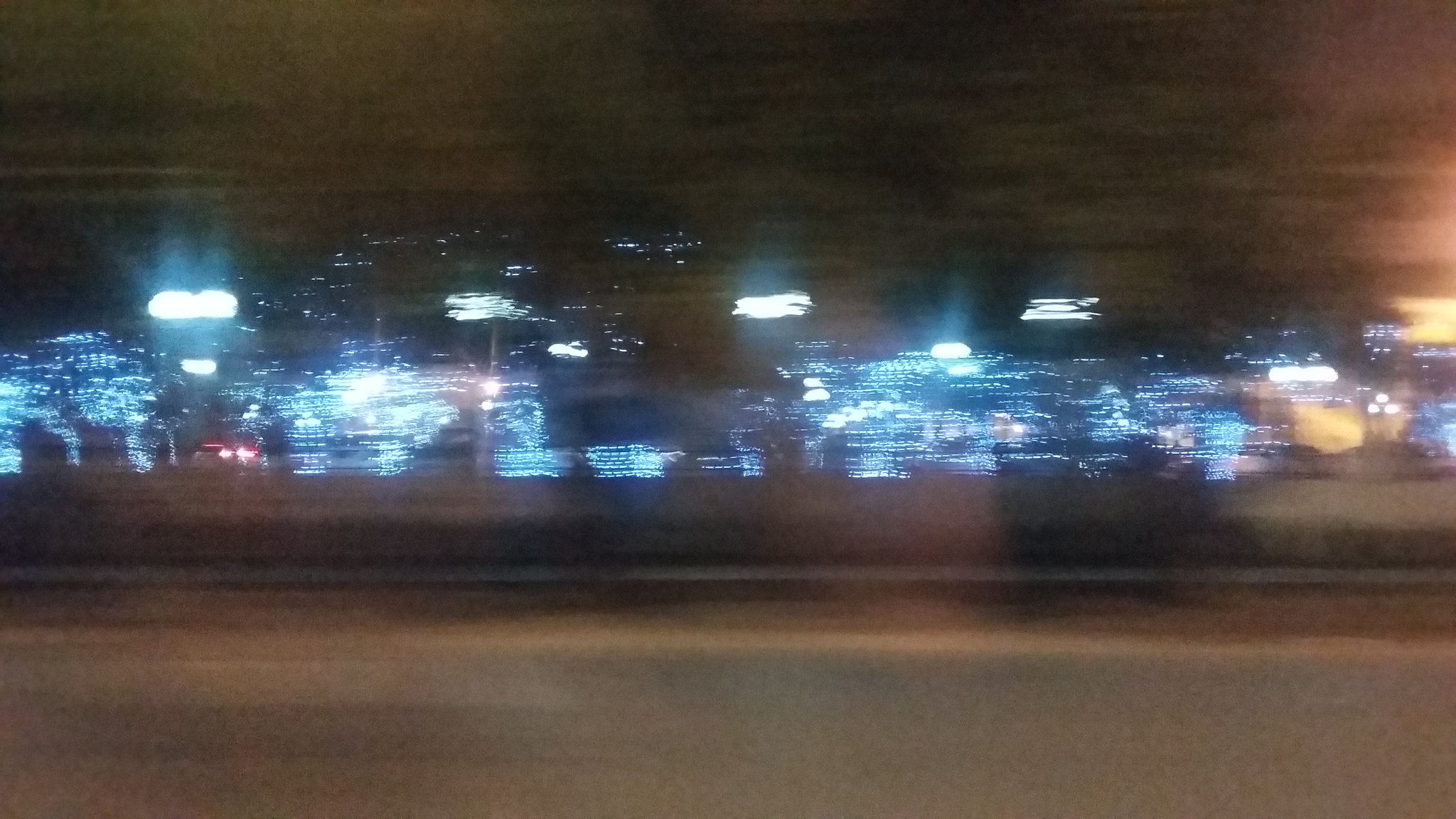A blurred nighttime photo captures the essence of a bustling cityscape, likely taken from a moving vehicle, possibly the passenger side of a car, as it travels along a highway. The image, albeit blurry, highlights the bright city lights piercing through the darkness, indicating a major downtown area with numerous buildings. Among the city lights, two prominent lights stand out on the left side of the image, mounted atop a solitary building. This building features an additional large light below, adding to the bright, lively ambiance of the urban night scene. The surroundings suggest the vehicle might be on an elevated roadway or within a tunnel-like bridge, adding a unique perspective to the blurred city view.